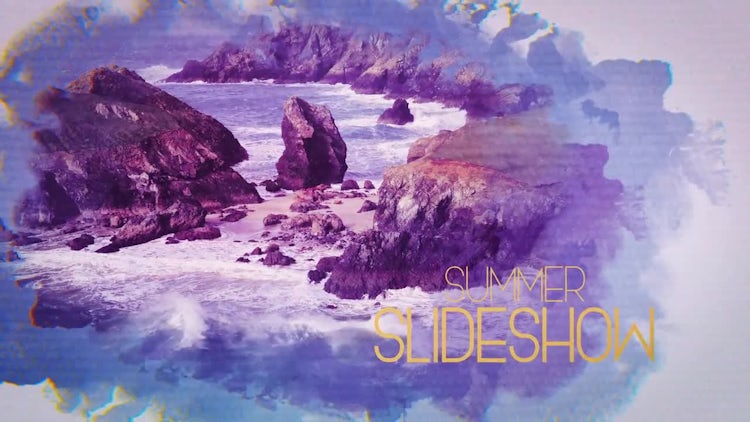This image, titled "SUMMER SLIDESHOW" in bold yellow letters, is an artistic portrayal resembling an airbrush painting. It prominently features a canyon with high, brown rock walls emerging from the ocean, forming a semi-circular formation. Waves are visible crashing against these rocky cliffs, producing white foam indicative of sea water. Nestled within this formation is a small, sandy beach with scattered rocks and a notable large boulder. The scene is encircled by a blue border, and the edges transition into a light gray backdrop with softer, whitish tones, creating a watercolor-like effect. The overall composition blends natural elements with an abstract, colorful overlay, capturing the vibrancy and dynamic essence of a seaside landscape.